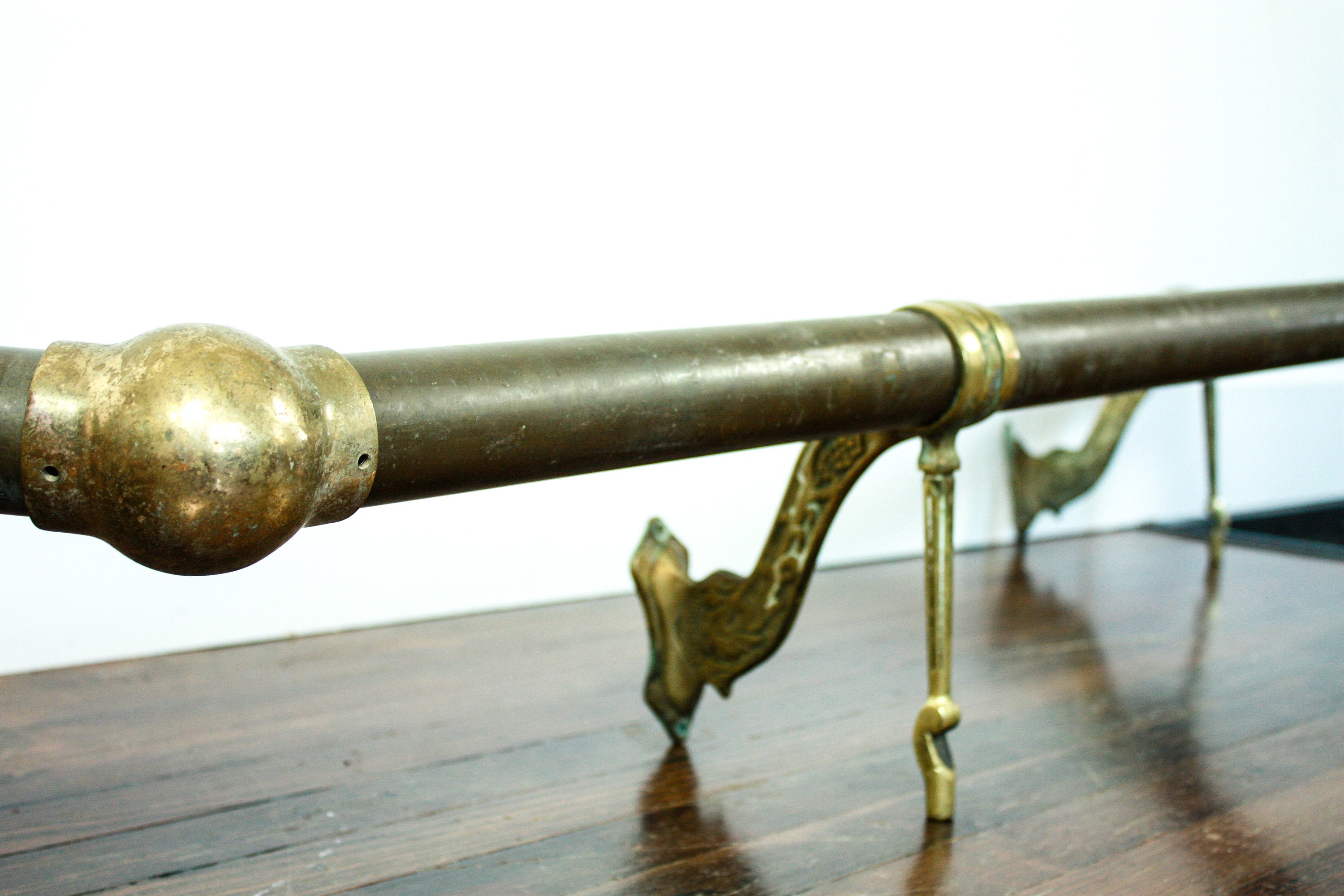In this color photograph, a detailed brass railing is displayed on a wooden horizontal paneled counter, possibly the top of a dresser or stand. The counter is comprised of lighter and medium-toned wood with some darker-toned wood and paneled strips, offering a rich, textured backdrop. The brass railing, positioned prominently across the center of the image, extends diagonally to the left and right.

At the left end of the railing, an elbow joint connects the horizontal bar to a vertical segment and includes a corner round piece with two small screw holes for securing it. Approximately halfway down, a central brace features a gold-toned straight peg as well as a curved, more ornate designed piece that serves as a stand, resting on the counter. A similar stand is visible further back in the image near the wall. The detail and reflection of the brass in the wood enhance the overall aesthetic, highlighting the craftsmanship of both the wood and the brass elements against a clean, white background.